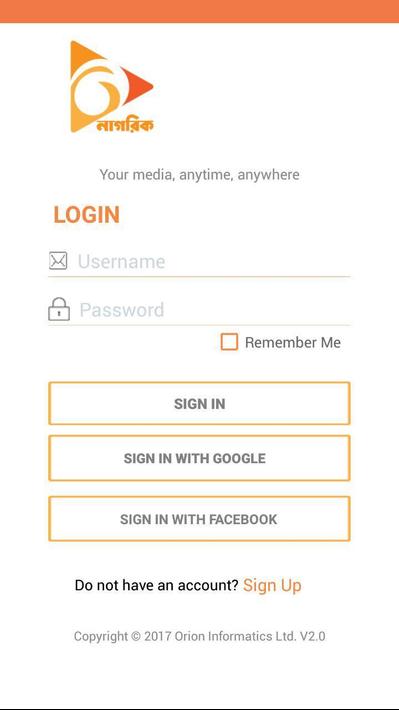This screenshot showcases a login menu from a website. At the very top, there's a prominent red navigation bar. Below this is the main login interface, which is set against a clean, white background. Immediately beneath the red bar, there's an icon reminiscent of the AOL symbol. Under the icon, there's text in a non-English, Asian language script. Below this, in gray font, it reads: "Your media, anytime, anywhere."

Prominently displayed in red, large, bold font is the word "Login." Directly below are two fields: one for entering a username and the other for a password. Beneath these fields, there's a small red checkbox accompanied by the text "Remember me" in black font. Further down are three outlined rectangles with red borders and white centers. The first rectangle contains the text "Sign In" in black font; the second reads "Sign In with Google" in black font; and the third, "Sign In with Facebook" in black font.

At the bottom of this page, in black font, it says "Do not have an account?" followed by "Sign Up" in red font. Finally, at the very bottom, the page is marked with the text "Copyright 2017."